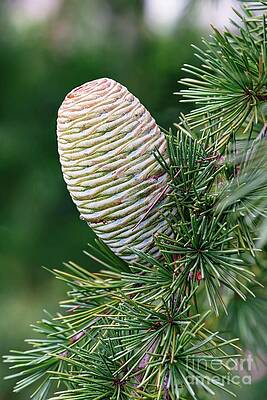The photograph, a vertical rectangular image, depicts a close-up of a branch from an evergreen tree, possibly a pine. The branch, adorned with numerous soft, pointed green needles, stretches diagonally from the upper right-hand corner towards the lower left-hand and lower right-hand corners of the frame. Prominently featured at the center of the image is an unusual, immature pine cone, about an inch high and less than a quarter inch wide, with smooth, circular, white, and light green horizontal striations. This oblong object, somewhat resembling a twisted ball of string or even a beehive, stands out against the blurred background of green trees and hints of gray sky at the top. The emphasis is on the striking contrast between the intricate pine cone and the soft focus of the surrounding foliage. Notably, in the lower right-hand corner, the text "Fine Art America" is visible, marking the photograph's source.